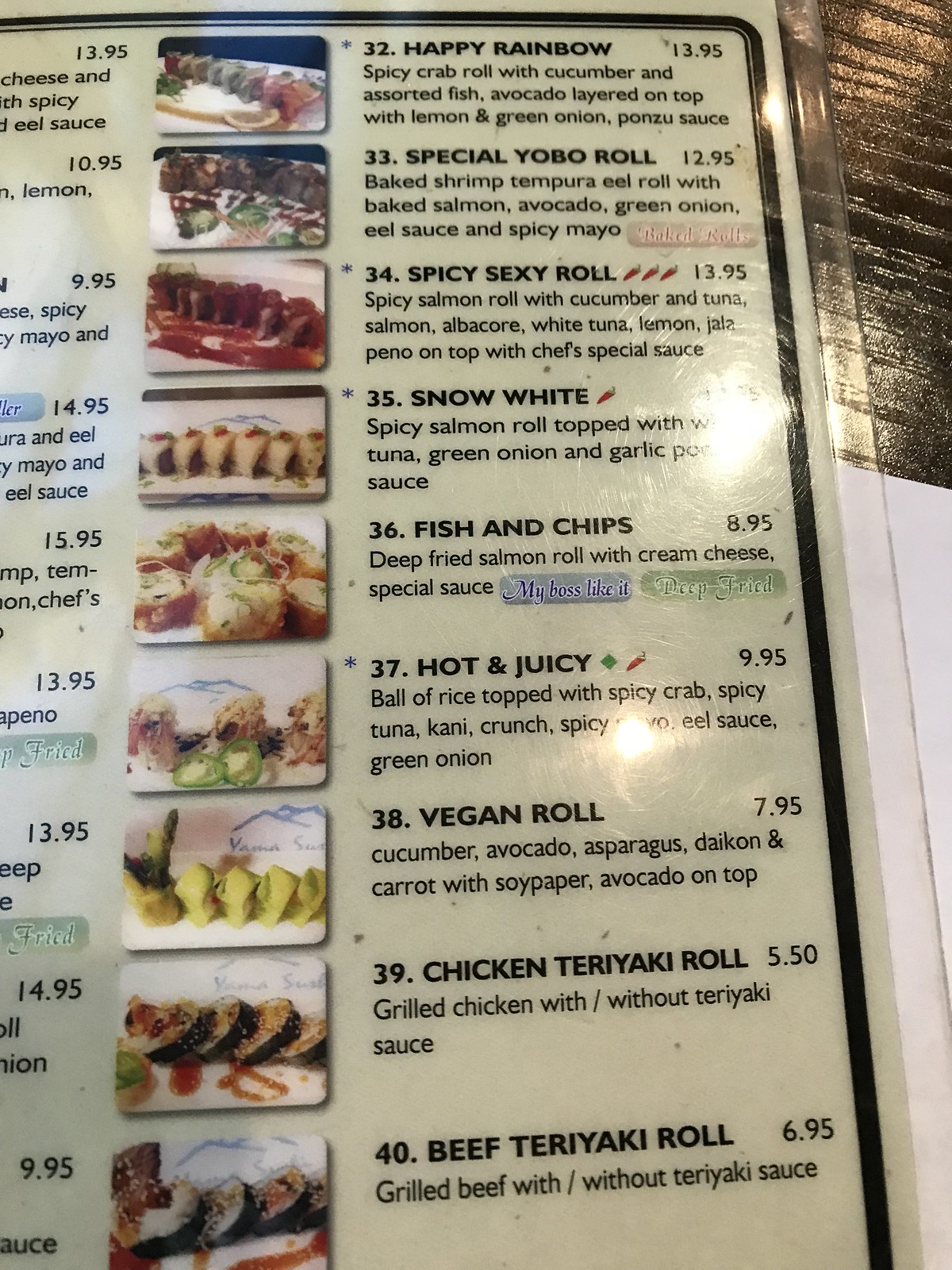**Detailed Caption:**

This close-up image captures approximately 60% of a laminated menu page from what appears to be an Asian restaurant, likely characterized by intricate and unique menu items. The menu, encased in clear laminate for easy cleaning, is predominantly a whitish-green color with a black border outlining the page. Given the occasional unusual phrasing, it seems the menu may have been created by someone for whom English is a second language. The descriptions resemble ingredient lists rather than evocative dish explanations.

The visible portion of the menu showcases items numbered 32 through 40, each accompanied by its price:

- **Happy Rainbow** ($13.95): Spicy Crab Roll with Cucumber, Assorted Fish, Avocado layered on top, Lemon, Green Onion, and Ponzu Sauce.
- **Special Yobo Roll** ($12.95): Baked Shrimp Tempura Eel Roll with Baked Salmon, Avocado, Green Onion, Eel Sauce, and Spicy Mayo.
- **Spicy Sexy Roll** ($13.95) denoted with three chili peppers: Spicy Salmon Roll with Cucumber, Tuna, Salmon, Albacore, White Tuna, Lemon, and Jalapeno slices on top, drizzled with Chef's Special Sauce.
- **Snow White Roll** ($13.95), indicated with one pepper for mild spice: Spicy Salmon Roll topped with Tuna, Green Onion, and Garlic Sauce.
- **Fish and Chips Roll** ($8.95): Deep-Fried Salmon Roll with Cream Cheese, and a blend of Special Sauce named 'My Boss Like It.'
- **Hot and Juicy Roll** ($9.95), symbolized with a green diamond and a red chili pepper: Rice topped with Spicy Crab, Spicy Tuna, Crunchy Tempura Bits, Spicy Mayo, Eel Sauce, and Green Onion.
- **Vegan Roll** ($7.95): Cucumber, Avocado, Asparagus, Daikon, and Carrot wrapped in Soy Paper, topped with Avocado.
- **Chicken Teriyaki Roll** ($5.50): Grilled Chicken with an option for Teriyaki Sauce.
- **Beef Teriyaki Roll** ($6.95): Grilled Beef, also available with or without Teriyaki Sauce.

Although the restaurant's location and specific Asian cuisine category remain unidentified, the array of dishes and eclectic combination of ingredients suggest a fusion of traditional and contemporary flavors.